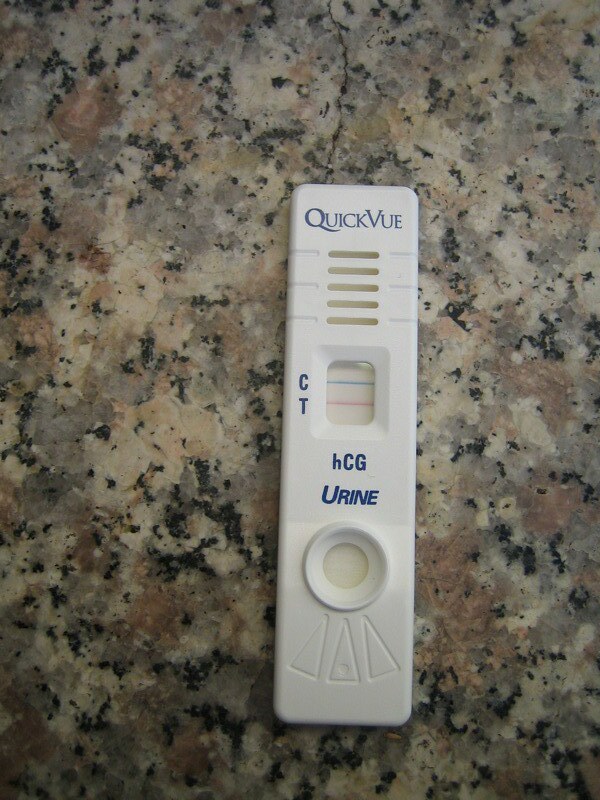The image depicts what appears to be a pregnancy test placed on a marble countertop that features a speckled pattern in black, white, and reddish hues. The rectangular plastic test device is white and prominently displays the brand name “QuickVue” (spelled Q-W-I-C-K-V-U-E) at the top in blue text. The test includes two distinct windows: one is rectangular with two visible lines—one blue (marked with “C”) and one pink (marked with “T”)—indicating the control and test lines, respectively. Beneath this window, the label “HCG” is written in blue text, with lowercase 'h' and capital 'CG,' followed by the word “urine.” There is an additional circular window below, whose purpose is not clearly indicated.